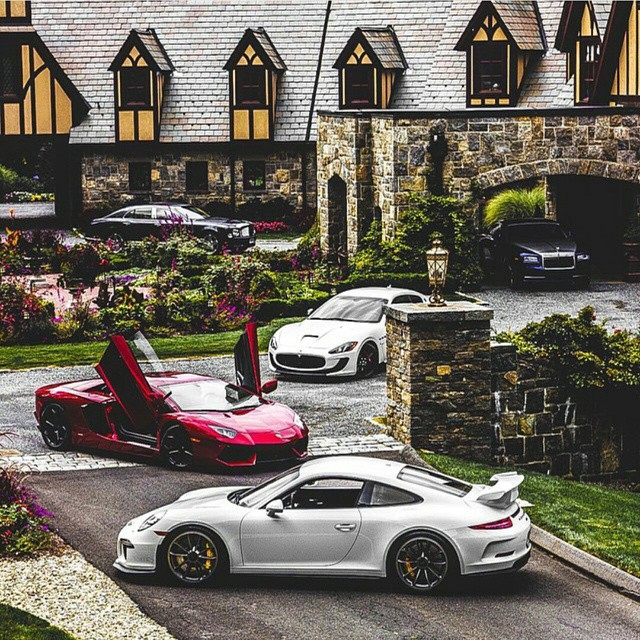This image showcases the lavish exterior of a stately old English manor, exuding an air of grandeur and opulence. The building, constructed with large stone bricks and adorned with six dormer windows, features a light tan roof, possibly slate, adding to its historic charm. A stone portico graces the entrance, sheltering one of the five luxury cars depicted in the scene.

The meticulously maintained grounds are lush with greenery and brimming with an array of vibrant flowers, including fuchsia plants. In the foreground, prominently displayed are three luxurious cars: a white Porsche with a distinctive rear fin, a sleek red Lamborghini with its flip-up doors open, and another white vehicle. Closer to the grand stone manor, partly obscured by the portico, sits a black car, while another black car rests further in the background. The assembly of vehicles includes models like Porsches and potentially Ferraris, Bentleys, or Rolls Royces, each adding to the overall sense of wealth and sophistication conveyed by the scene. The setting, with its dark, rich coloring, evokes a timeless elegance, making the mansion appear as a quintessentially high-end estate.